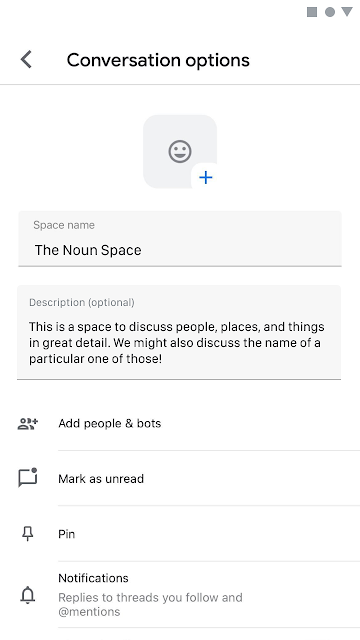The image features an interface layout on a white background. At the top, there is a gray square with a smiley face and a blue plus symbol. Directly below this, there's a section titled "Conversation Options" with a left-pointing arrow beside it. Below this title is a horizontal gray line, and above it to the right are three icons: a square, a circle, and a downward-pointing triangle.

Underneath the smiley face icon, there's a gray rectangular text box labeled "Space Name (Noun)." Below this text box is a larger gray rectangular area labeled "Description (Optional)" which provides a prompt: "This is a great space to discuss people, places, and things in great detail. We might also discuss the name of a particular one of those."

Further down, the text "Add People and Bots" appears above a light gray horizontal line. Below this line, the text "Mark as Unread" is displayed, followed by another light gray line. Next, there's a pin icon to the left of the text "Pin," with yet another light gray line underneath. Additionally, there's a notification bell icon accompanied by the text "Notifications: Reply to threads you follow and mentions," wrapping up the interface details with a final horizontal gray line at the bottom.